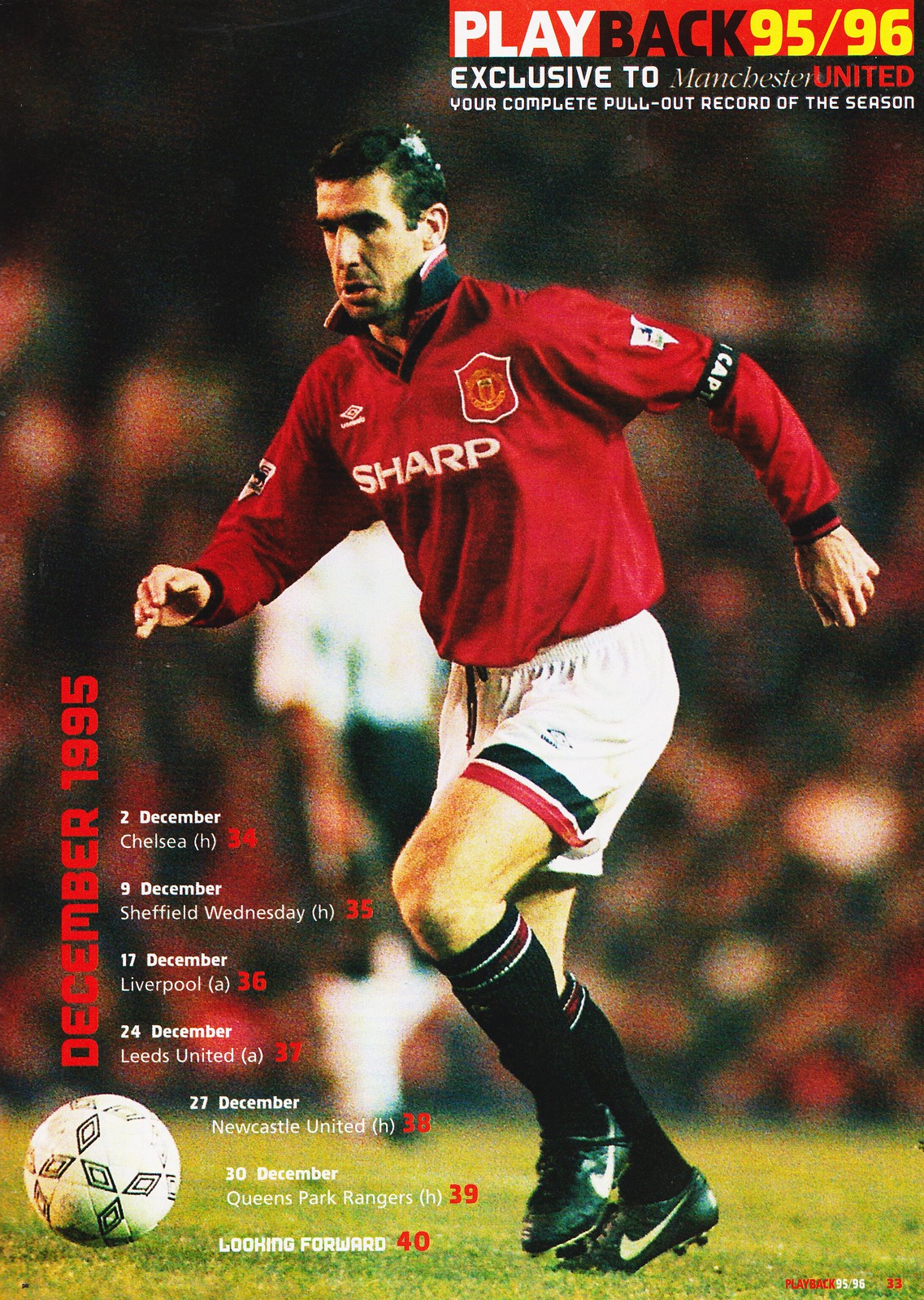The magazine cover for an English football club is a vivid depiction of a soccer event advertisement. Prominently featured in the center of the cover is a soccer player with short black hair. He's mid-action, with arms outstretched, one forward and one backward, a knee bent in front, and one foot slightly off the ground as he runs towards a white soccer ball with black decals situated in the bottom left corner. He wears a vibrant red long-sleeved top with the word "sharp" emblazoned in white across the chest. His blue shorts have circular logos—one black and one red—just above the knees, and he is equipped with black knee-high socks and black Nike cleats marked with white swooshes.

The background captures a blurred crowd, emphasizing the player’s dynamic movement on the green field. In the upper right corner of the cover, against an orange backdrop, the text reads "Playback 95-96 Exclusive to Manchester United. Your complete pullout record of the season." Vertically aligned, in the bottom left corner, the date "December 1995" appears in red text. Adjacent to it, a detailed schedule lists upcoming matches: “2 December Chelsea, 34; 9 December Sheffield Wednesday, 35; 16 December Liverpool, 36; 23 December Lettsfield, 37; 27 December Newcastle United, 38; 30 December Queen's Park Rangers, 39; 31 December Lohingford, 40."